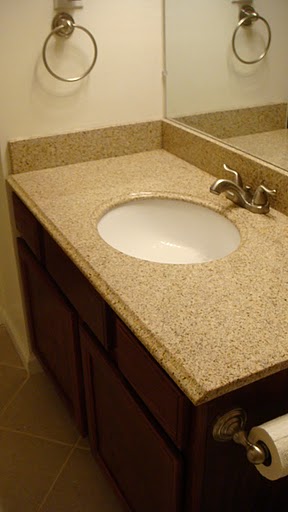This image depicts a meticulously organized bathroom sink area. The countertop exudes a tan, sandy appearance, reminiscent of gritty beach sand, though it is smooth to the touch. The sink basin is a pristine white, complemented by a gleaming silver faucet. Behind the sink, a mirror captures the reflection of the sandy countertop, adding depth to the scene. To the left of the sink, a sleek silver hoop wall mount holds a washcloth or hand towel within easy reach. 

The cabinets beneath the sink are a rich, dark brown, providing a striking contrast to the lighter countertop. The flooring underfoot is a blend of brown tiles with white grout, which ties the earthy tones of the room together. On the right side of the image, part of a toilet paper roll is visible, affixed to the side of the sink cabinet with a matching silver holder. The white toilet paper and its holder echo the silver accents found throughout the bathroom. The light in the room casts subtle glares on the metallic elements and the countertop, adding a touch of sparkle to the serene space.